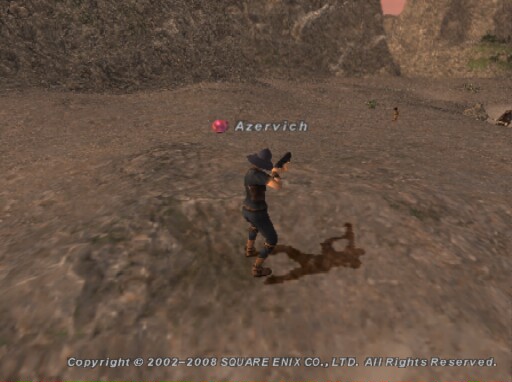This detailed color image, a screenshot from the game Final Fantasy XI, captures a character named Kazurvich, a figure prominently positioned in the middle. The character casts a shadow to the right and appears to be standing on a gravelly, grainy, brown rocky surface—indicative of a desert-like terrain, possibly the North Gustaburg area. The character, rendered with light skin, is outfitted in a black rain cap resembling a pirate or military hat, black leather pants, sandals, a black vest, and brown boots. He is armed with a low-level black gun aimed at a distant, tiny ground worm. Above his head, a red dot and his name "Kazurvich" or "Azarevich" is displayed in white lettering. The bottom of the image clearly features a copyright stamp: "Copyright 2002-2008 Square Enix Co., Ltd., All Rights Reserved." This image highlights the game's meticulous design and the legacy of Final Fantasy XI, a title that remains online despite its age.